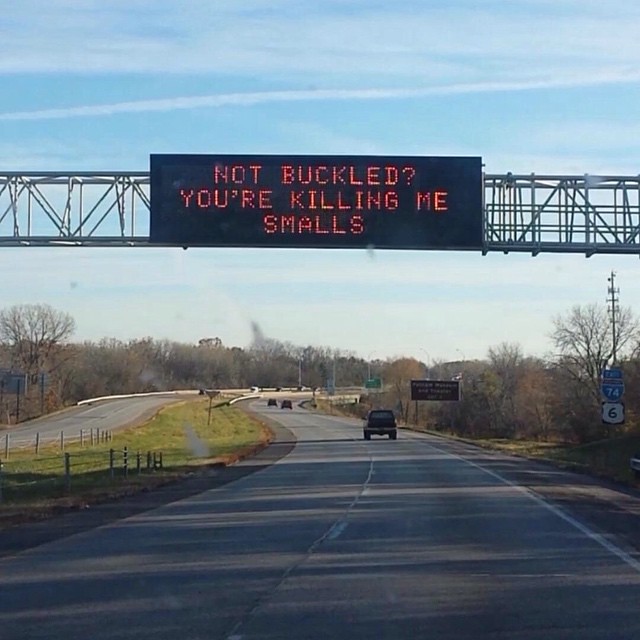This detailed photograph captures a divided interstate highway with a grassy median. The highway features two lanes in each direction, lined by a mix of deciduous trees that have shed their leaves, indicating it is likely late fall or early spring. The sky occupies the upper two-thirds of the image, dotted with some clouds. Multiple vehicles, including a truck and at least three cars, are visible, both oncoming and moving away.

A prominent feature of the scene is a digital LED sign mounted on metal scaffolding overhead, displaying a humorous and cautionary message in red text: "Not Buckled?" on the first line, "You're Killing Me," on the second line, and "Smalls" on the third line. This sign hangs above the roadway, drawing attention to the importance of seatbelt usage.

Alongside the road, on the right-hand side, there is a highway sign with a blue shield indicating "East 74" and another shield with black numbers indicating "6." The highway curves gently to the left and then sweeps sharply to the right in the background. A brown highway sign in the far distance announces an undetermined destination, adding to the depth and context of the scene. The photograph appears to be taken from a moving vehicle, capturing the essence of a cold season highway journey.